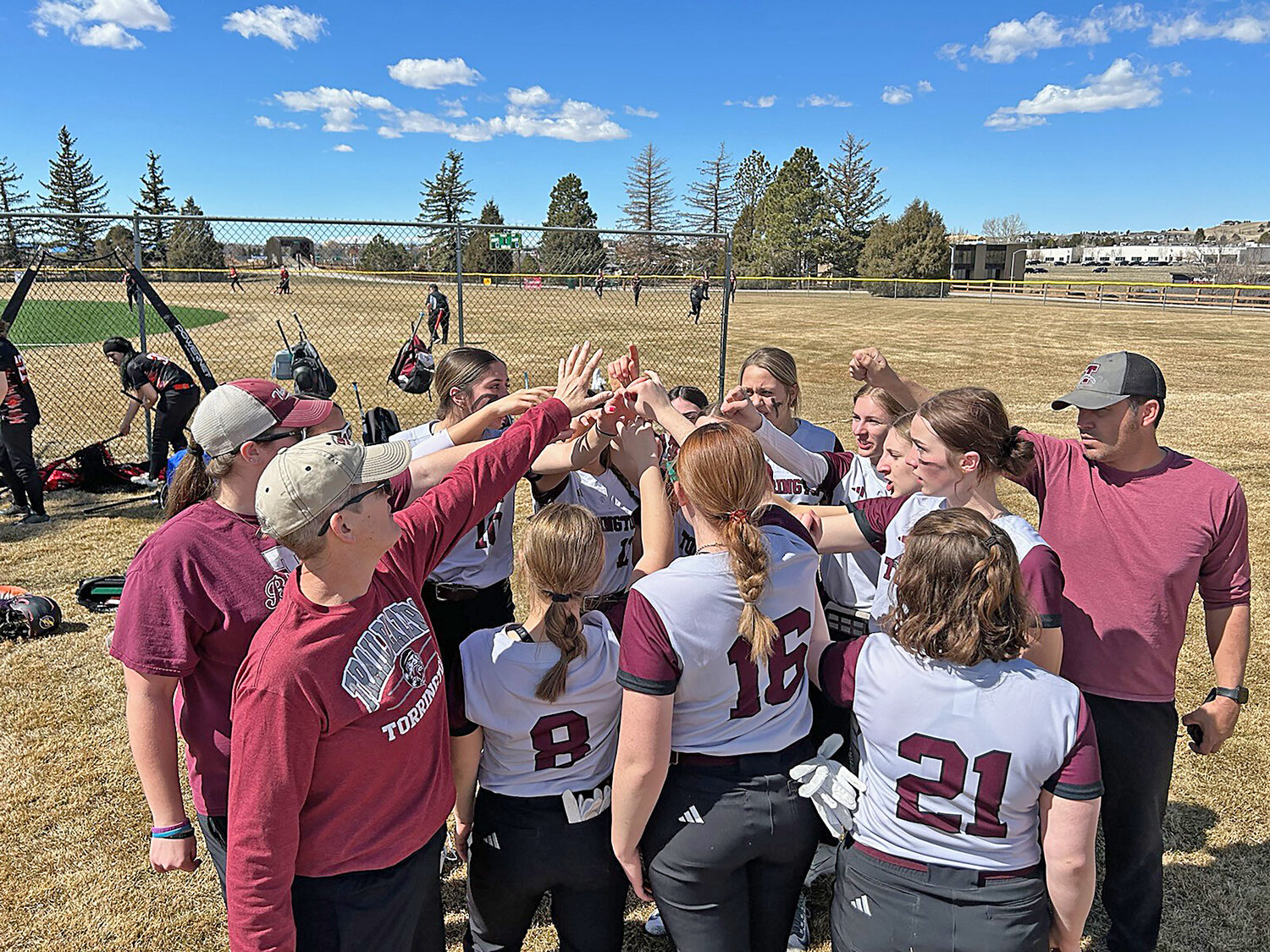In this photograph, a female softball team is captured either just before or just after a game, all joining hands in a gesture of unity and encouragement. The team consists of 10 players, all females, and is accompanied by two female coaches and one male coach. They are standing on a dry, brownish-yellow field under a blue sky scattered with white clouds. The players, wearing white shirts with maroon sleeves and numbers, as well as black adidas pants, have their hair styled variously up or down, with three of them donning hats and all sporting black face markings.

In the background, the scene reveals a typical softball field bordered by a wire fence, with trees that lack full foliage, suggesting the season could be fall or winter. Further back, there are several buildings partially visible and another team on the left-hand side appears to be packing up their gear. Noteworthy details include the numbers 8, 16, and 21 on the backs of three players facing away from the camera. The atmosphere conveys a sense of camaraderie and readiness, as the team prepares for or celebrates their game.